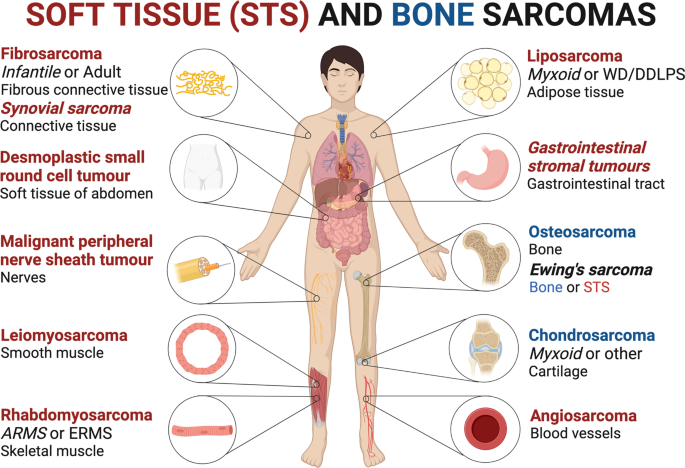This is a highly detailed medical diagram titled "Soft Tissue (STS) and Bone Sarcomas," presented at the top in red and black text. The central illustration features the anatomical body of a light-skinned male, depicted in a lifelike manner with various internal organs, tissues, and bones visible. The skin is illustrated in light tones, the stomach and outer stomach marked in shades of pink, kidneys in brown, veins in blue, and the trachea also in blue.

Circles and call-out arrows surround the body, magnifying and detailing specific regions where different sarcomas are located. The diagram highlights and labels multiple types of sarcomas, including:
- Fibrosarcoma (left shoulder)
- Synovial Sarcoma
- Desmoplastic Small Round Cell Tumor (abdomen)
- Malignant Peripheral Nerve Sheath Tumor (thigh)
- Leiomyosarcoma (shin)
- Rhabdomyosarcoma (shin)
- Liposarcoma (shoulder)
- Gastrointestinal Stromal Tumors (gastrointestinal tract)
- Osteosarcoma (right leg bone)
- Chondrosarcoma (right leg cartilage)
- Angiosarcoma (blood vessels in lower leg)

Each sarcoma is identified with magnified circular images and call-out lines elaborating on the specific tissue or bone area affected. Definitions and detailed descriptions are placed to the left and right sides of the body, with some text in red to enhance visibility. This comprehensive diagram, which appears to be from a medical journal or webpage, serves as an educational tool detailing the various soft tissue and bone sarcomas evident within the human anatomy.